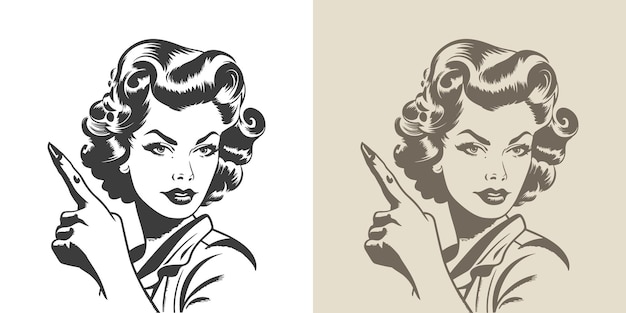The image is a side-by-side comparison of two black-and-white sketches of the same woman, with one drawing on a white background and the other on a light cream or tan background. The sketches show the woman from just below her shoulders up, featuring short, curly hair that hits just over her ears, a mix of black and white strands. Her eyebrows are distinctly arched and dark, complementing her large, expressive eyes adorned with heavy mascara. She gazes slightly down and to the right, her lips dark and slightly parted, hinting at possible reflections or a glimpse of her teeth. She has an angular, youthful face that suggests she may be in her 20s or early 30s. The woman's left hand is raised to her chin with a long, sharp fingernail pointing upward and leftward, highlighted by a black circle over her knuckles. She wears a collared shirt, and the area beneath her chin is shaded in black to create a shadow, adding depth to the portrait.